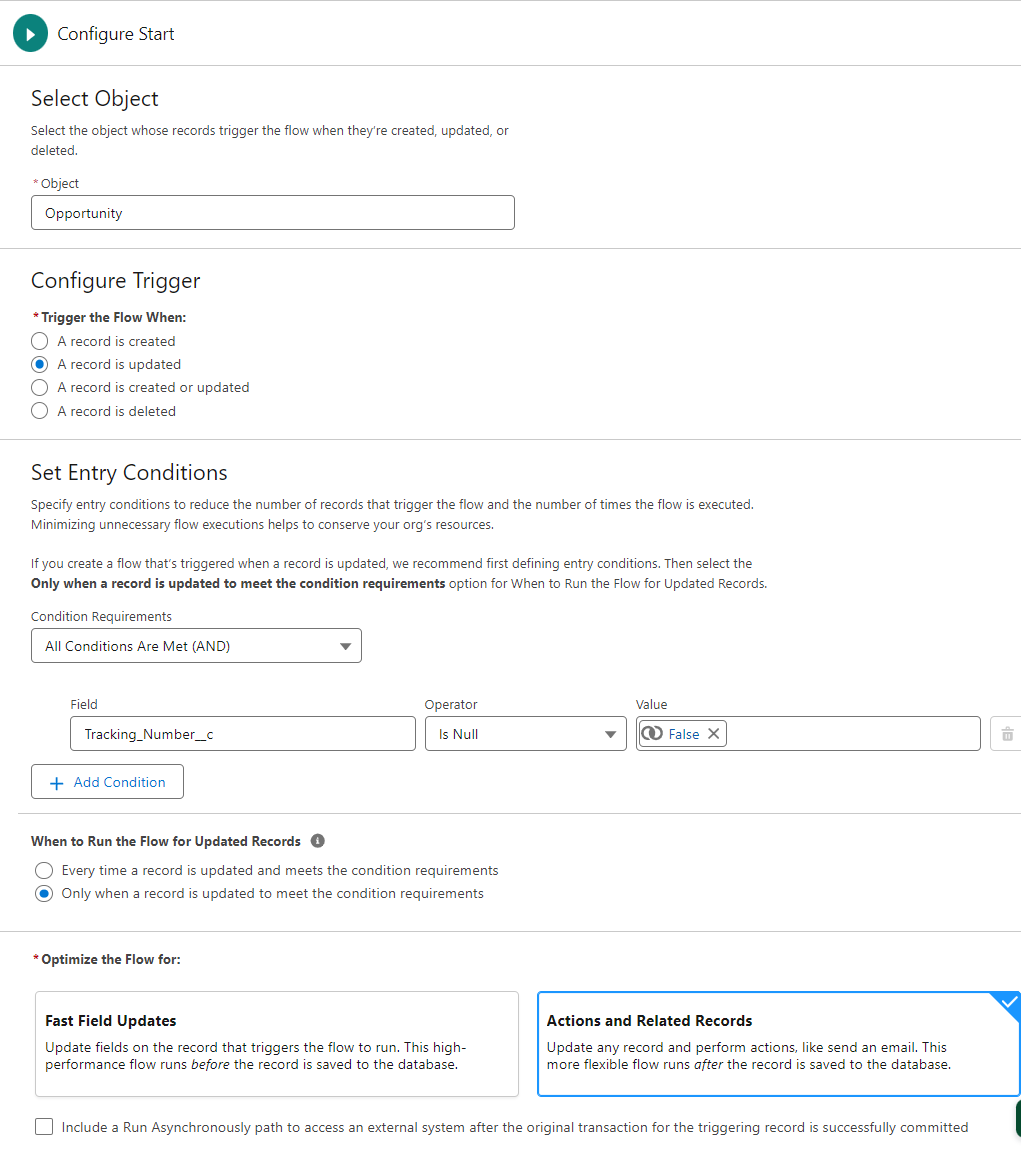This image is a detailed screenshot from a configuration section of a website. At the top center, the heading "Configure Start" is prominently displayed with both "C" and "S" capitalized. 

On the left side, the section begins with "Select Object" followed by the description “Select the object whose records trigger the flow when they're created, updated, or deleted.” Below this, the term "Object" is marked with a red asterisk, indicating a required field. Adjacent to it, a dropdown box displays the option “Opportunity.” 

The next segment, titled "Configure Trigger" in bold text, contains another red asterisk. It prompts the user with "Trigger the flow when" and presents four options: "A record is created," "A record is updated," "A record is created or updated," and "A record is deleted." In this instance, the option "A record is updated" is selected.

Continuing downward, the section "Set Entry Conditions" includes several paragraphs that are not fully visible. It specifies "Condition Requirements" with the criteria "All conditions are met." 

The conditions detail that the "Field" is "Tracking Number," the "Operator" is "Is null," and the "Value" is "False." There is also a blue button labeled “Add Condition.”

Further down, the section "When to Run the Flow for Updated Records" offers two choices: "Every time a record is updated and meets the condition requirements," or "Only when a record is updated to meet the condition requirements." The chosen selection here is "Only when a record is updated to meet the condition requirements."

Finally, the section titled "Optimize the Flow for" is marked with a red X right before it, indicating perhaps an incomplete selection or an error.